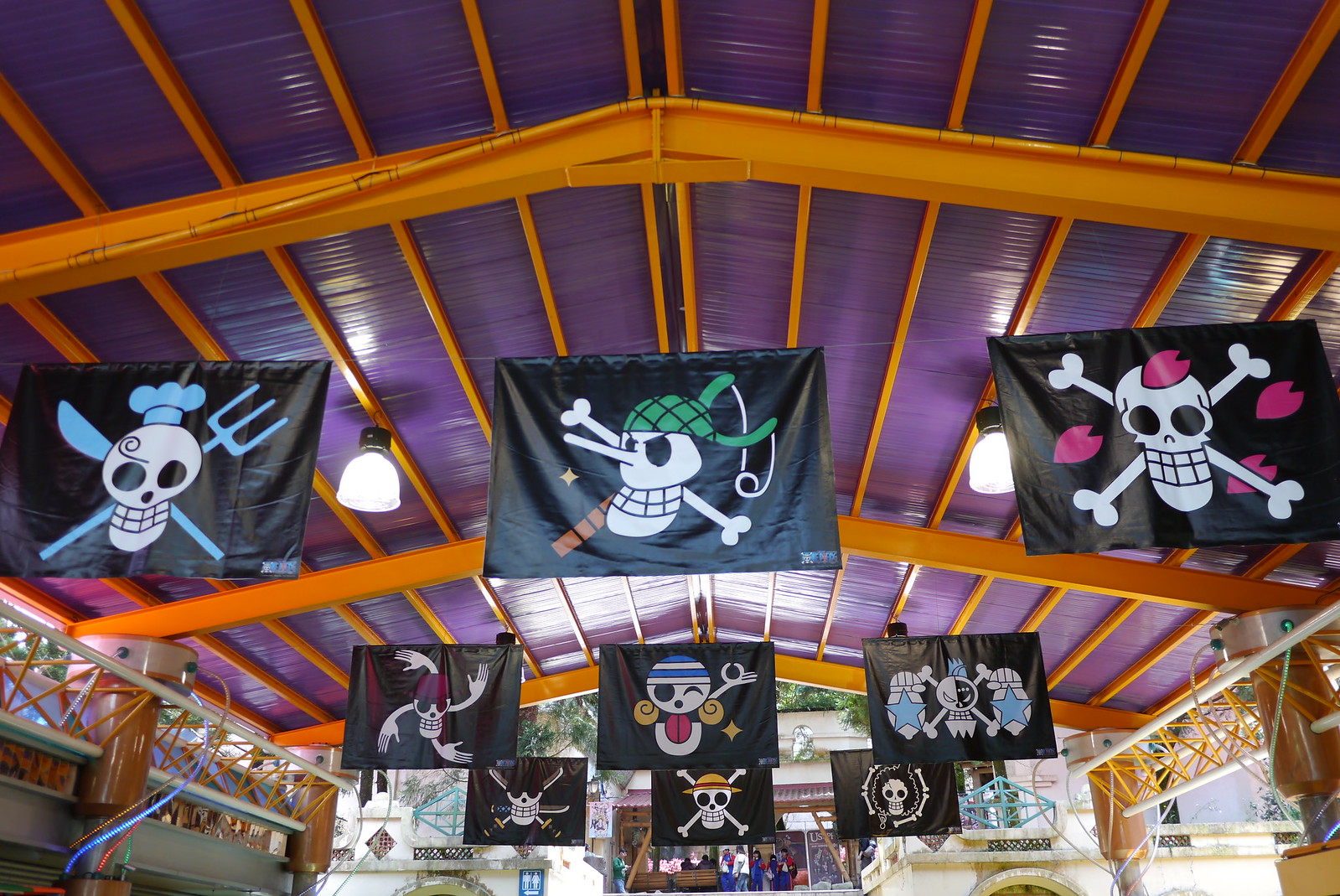The photograph captures an angled upward view of a makeshift canopy structure over a street market stall, possibly located in a theme park or amusement park. The canopy is formed by bright pumpkin orange beams or rafters crisscrossing against an eggplant purple tarp that provides weatherproofing. On each side, there's additional beam and bar siding. Hanging from the ceiling are nine black background flags with various comical skull designs, ranging from a white skull with a blue chef hat and crossed fork and knife, to a skull encircled by red hearts, each design being more cartoonish and crafty. Additionally, two lights dangle from the ceiling. At the bottom of the image, the tops of market stalls can be seen to the left, a bathroom sign in the center, and some distant people and buildings further back, giving a lively and bustling ambiance.